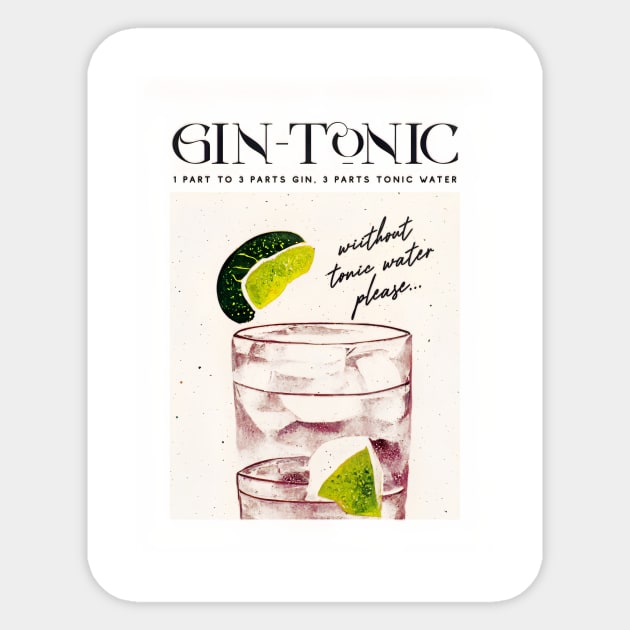The image is a vertically rectangular advertisement for a gin and tonic recipe. The outer background is gray, with a white inner rectangle that has rounded corners, creating a clean and modern look. Inside this white frame, there's a smaller pink rectangular box with digital and cursive text. At the top, bold and fancy capital letters spell out "GIN-TONIC." Below this title, in smaller but still capitalized text, the proportions for the drink are listed: "One part to three parts GIN, three parts TONIC WATER."

Beneath the recipe instructions, in cursive script, it reads "without tonic water please...", adding a playful touch. The focal point of the advertisement is a clear glass filled with ice cubes and lime wedges; one lime wedge hovers above the glass, while another rests inside it. The glass appears to be a short tumbler, adding to the classic aesthetic of the drink's presentation. The overall design features a layered composition with a sophisticated yet approachable vibe, likely intended for marketing purposes.